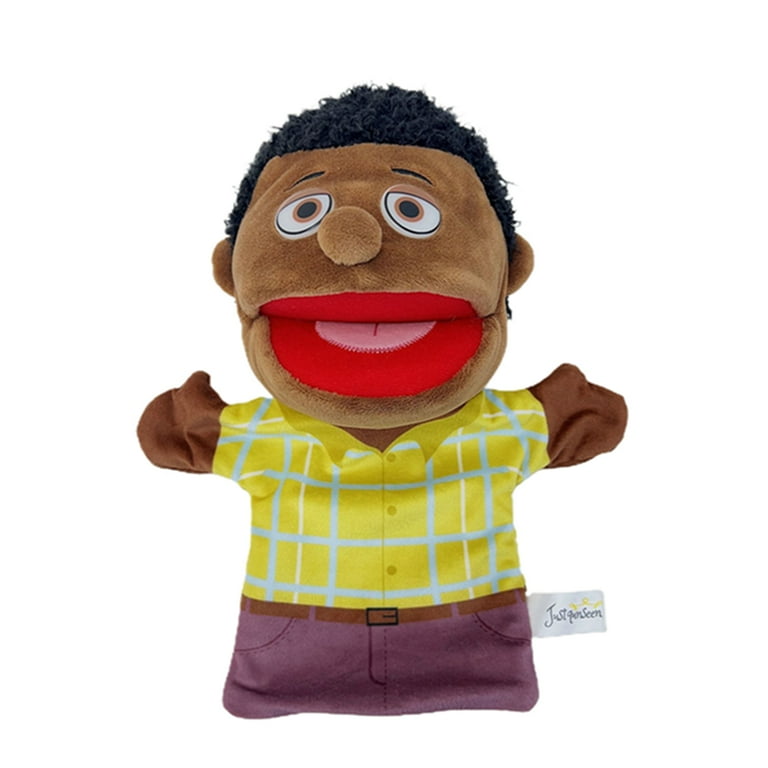The image features a child's hand puppet with Afro-Caribbean characteristics, designed in a cartoony style reminiscent of the Muppets. The puppet has short, black woolly hair, large expressive brown eyes, a wide open red mouth with a pink felt tongue, and a small brown pom-pom for a nose. It is dressed in a yellow shirt with turquoise checks, a little brown belt, and purple pants that only extend to the bottom of the crotch, giving it a square-shaped body. The puppet's hands are outstretched, protruding from the sides of its body. A tag on the puppet reads "Just Quinceine," possibly indicating the name or brand. The image has an all-white background, with the puppet lying flat center frame, emphasizing its playful and accessible design for children's use.